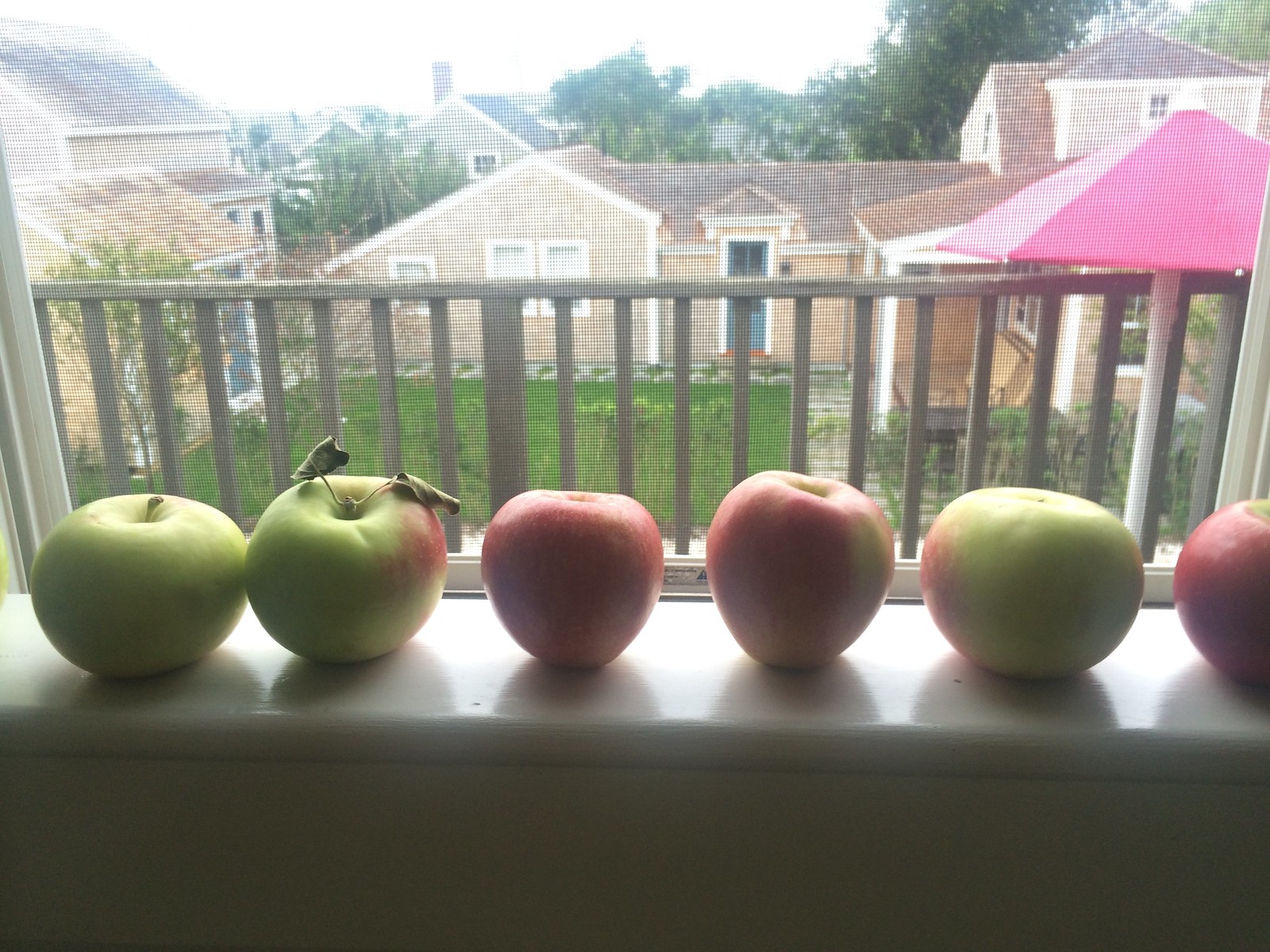This image captures a sunlit scene of six apples arranged on a white-painted windowsill within a screened window. The second apple from the left has a distinctive stem with two leaves. The apples display a vivid mix of colors: some are fully red, others are primarily green with hints of red. The apple furthest to the right is only partially visible. Beyond the window, you can see a small balcony with a gray railing and a pink umbrella, set amidst a well-tended yard. The yard features a stone walkway and manicured grass, with trees scattered around. In the distance, several houses can be seen, two of which have blue doors, all enveloped in bright daylight that washes out the sky. The overall scene exudes a tranquil, domestic charm with a hint of the bustling residential area beyond.